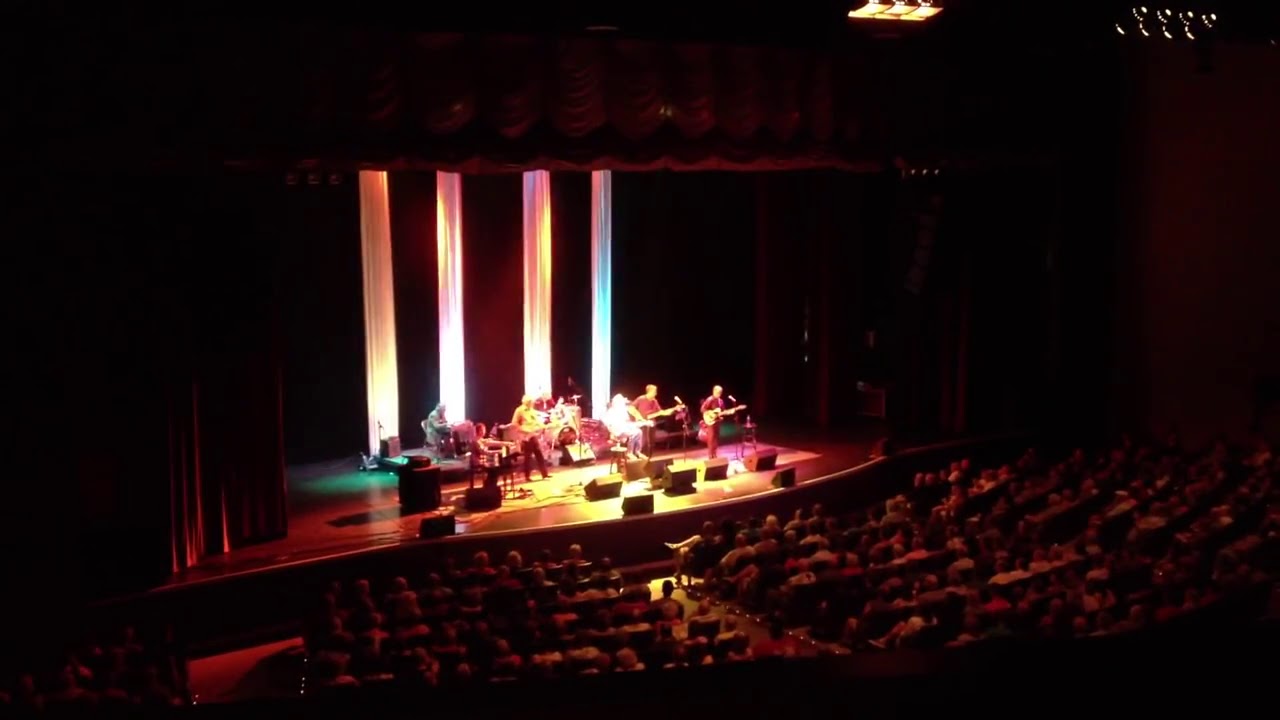This photograph captures the interior of a musical theater from an elevated vantage point. The image prominently features a wide, mahogany-colored wooden stage, well-lit and elevated above the audience. The stage is alive with approximately 10 to 12 musicians, including a drummer, two guitarists, a bass player, and possibly a keyboardist, all engaged in a performance. While most musicians are seated, a notable figure stands at the center, clad in brown pants and a yellow top. The surrounding areas of the theater are shrouded in darkness, with illumination concentrated on the stage.

The backdrop, bathed in a vibrant red lighting theme, consists of four vertical fabric strips in shades of orange, pink, and blue, adding a pop of color to the composition. Overhead, stage lights are faintly visible, especially near the upper right corner of the image.

In the foreground, rows of auditorium-style seating are filled with attentive audience members, their seats arranged in three visible sections. Curtains flanking the stage hint at their ability to close over the performance area, and dark surroundings emphasize the focus on the vibrant activities on stage.

Overall, the image conveys a dynamic, immersive experience of a musical performance within a darkened theater, highlighting both the musicians and the engaged audience.